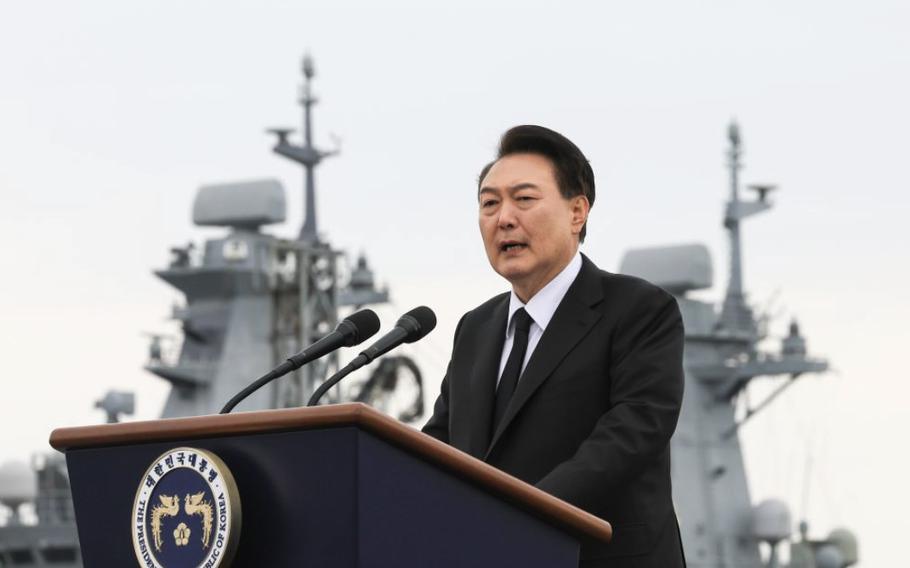This image captures an older Asian man, presumably of Korean descent, speaking at a podium on what seems to be a military vessel, likely an aircraft carrier. The man, who might be a high-ranking official or even the President of Korea, is dressed formally in a black suit, black tie, and white undershirt. His hair is short, black, and slightly curves to the right. He is addressing the audience through two black microphones mounted on stands, visible against the podium. The podium itself has a dark blue body with wooden trim and bears an emblem featuring Asian characters and symbols, including two sideways L-shapes with a flower between them, and the words "The Republic of Korea" in English below. Behind the speaker, the towering gray structures and antennae of a battleship can be seen, bathed in daylight. The man has his mouth open, mid-speech, contributing to the dynamic action of the scene.